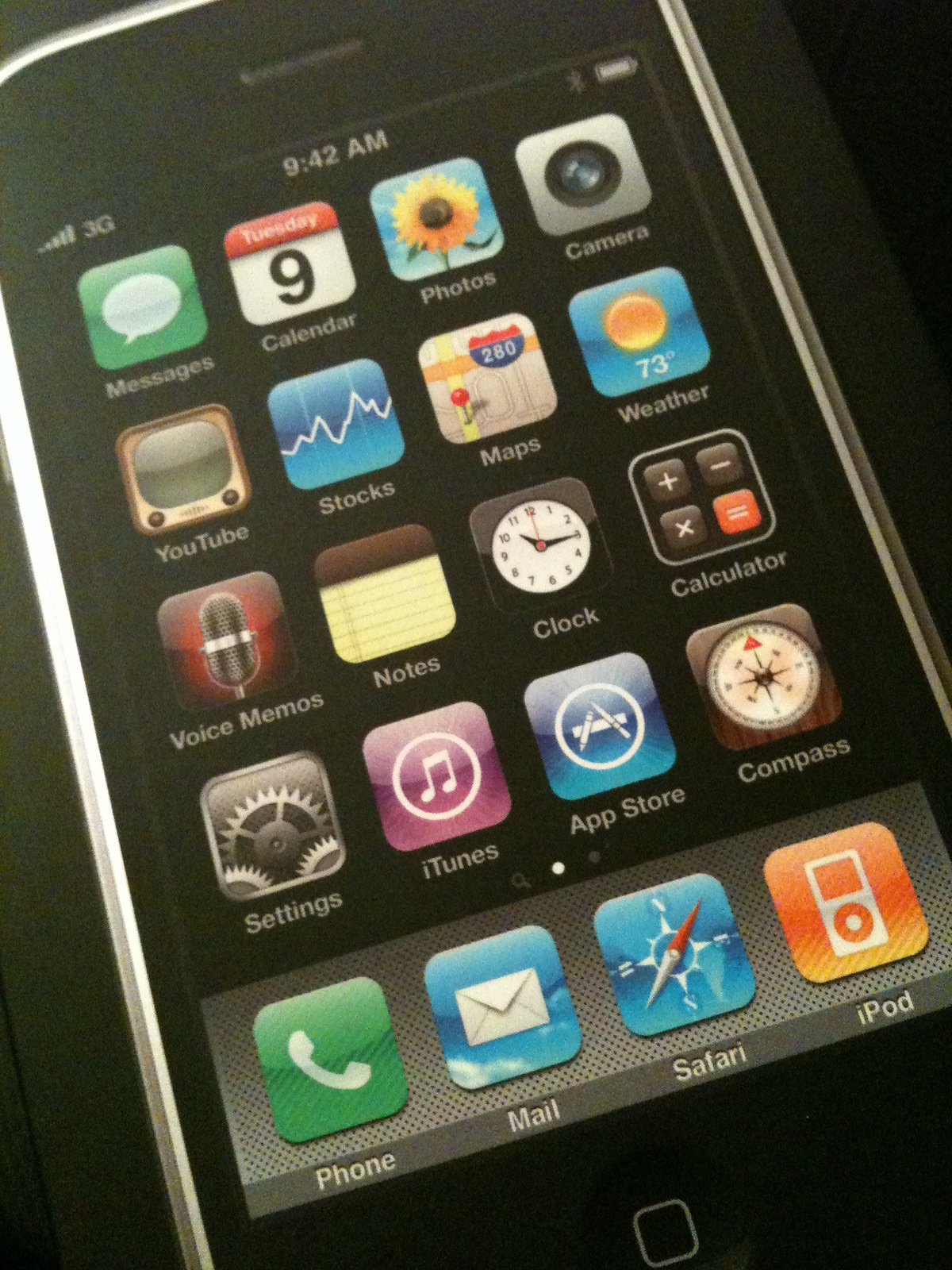The image depicts a classic black Apple iPhone, likely from around 2007 to 2009, displayed against a black background. The phone has a silver edge and a black screen. The device is slightly tilted to the left and shows the time as 9:42 AM with a filled battery bar and a 3G network indicator. The screen displays five rows and four columns of app icons, which include Messages, Calendar, Photos, Camera, YouTube, Stocks, Maps, Weather, Voice Memos, Notes, Clock, Calculator, Settings, iTunes, App Store, and Compass. The bottom row of the stationary dock features the Phone, Mail, Safari, and iPod icons. The phone's screen appears somewhat hazy, suggesting the image is either old or a photograph of a printed photo. This reinforces the impression of the device's vintage nature, reflective of the early iPhone models. The home button is visible as a rounded-corner white square in the center.